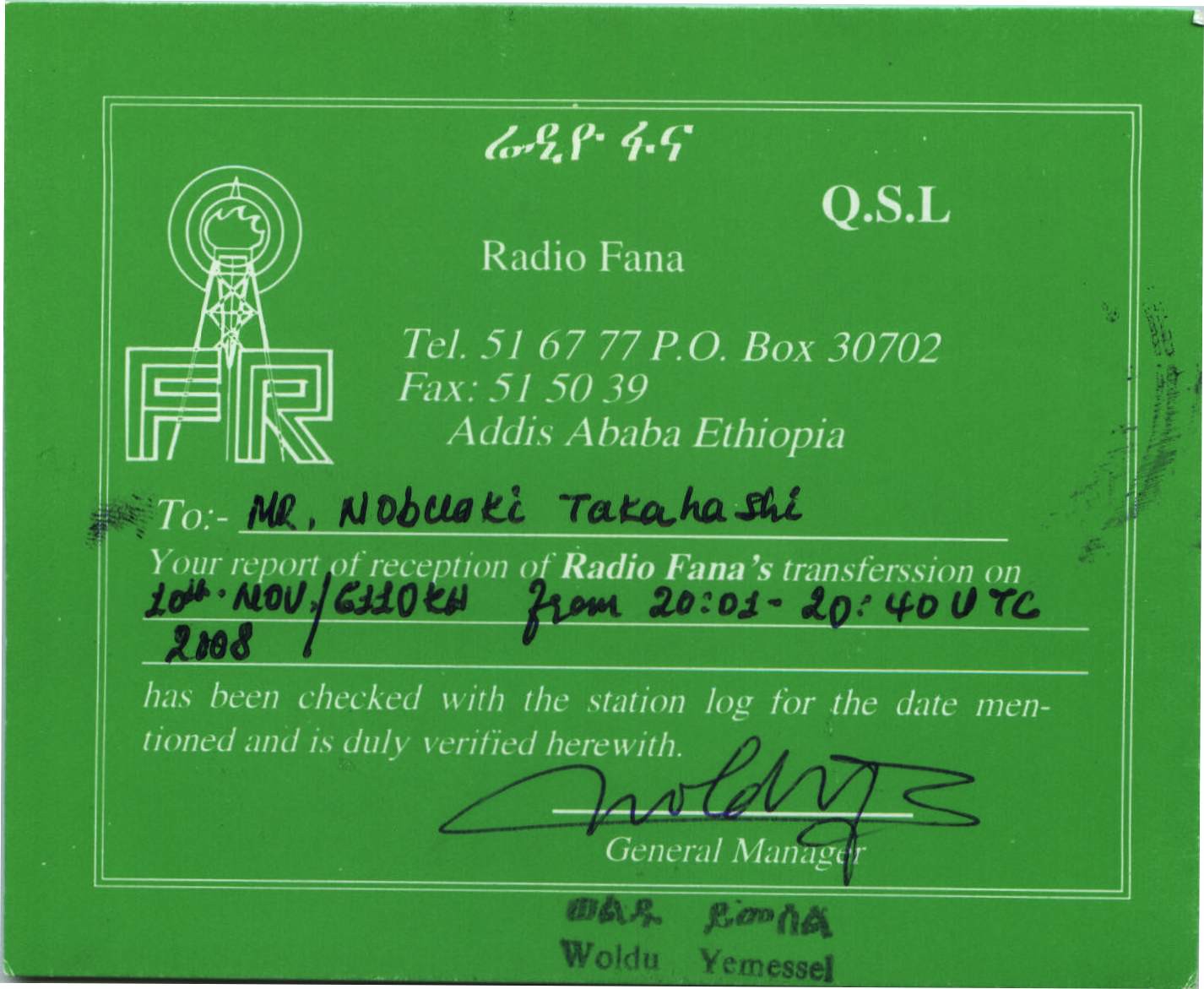The image displays a green certificate card with a white double border and detailed information both printed and handwritten. At the top, the card prominently features "Radio Fana" with a white illustration of a radio tower emitting signals in front of the letters "FR." Below this, the contact details are listed in white text: "Tel: 516777, P.O. Box 30702, Fax: 515039, Addis Ababa, Ethiopia." 

In the middle section, there's a field designated "To," with the handwritten name "Mr. Nabuaki Takahashi." Further down, white text states, "Your report of reception of Radio Fana's transversion on," followed by handwritten details, "20th November 6110 kHz from 2001 to 2040 UTC 2008." It continues, "has been checked with the station log for the date mentioned and is duly verified herewith."

At the bottom, there's a space for a signature which is filled in, identified as signed by the General Manager of Radio Fana. The certificate formally acknowledges the reception report, providing a verified confirmation in a detailed and official format.